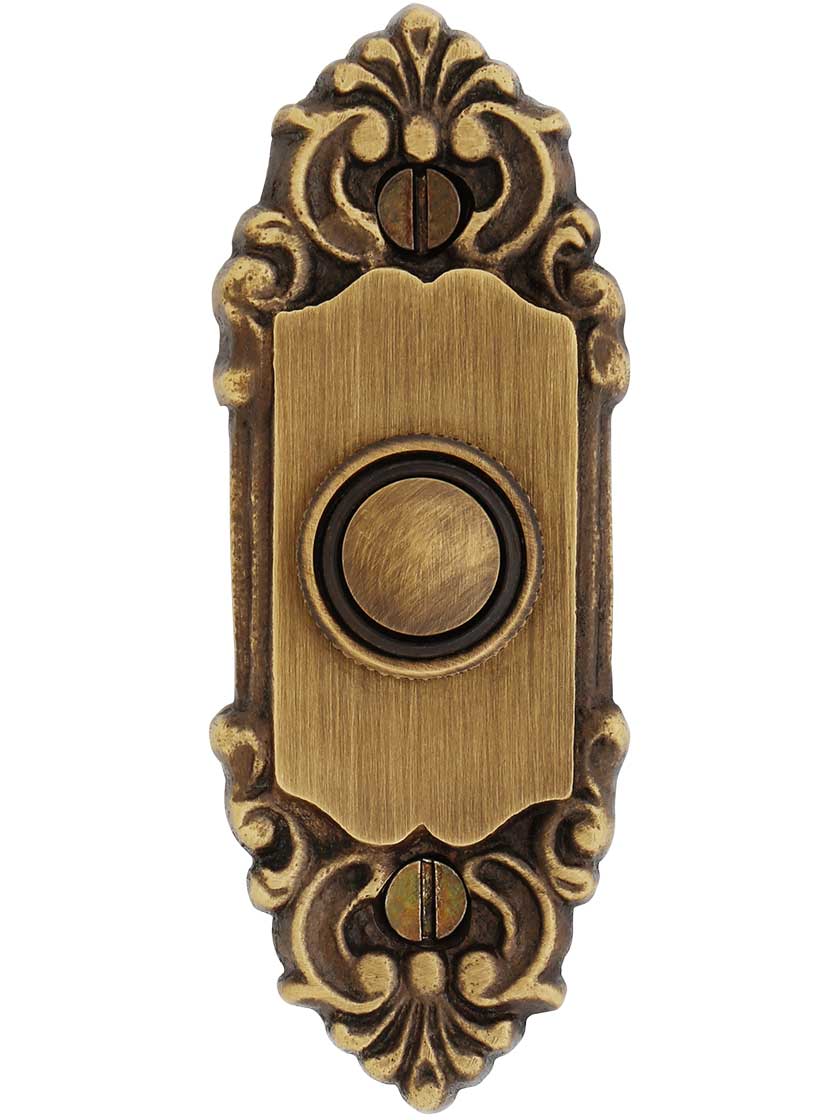This photograph features a vintage-style doorbell isolated from any background. The doorbell housing is made of brushed brass, imparting a slightly aged and weathered appearance with its gold and dark brown hues. The housing features an intricate floral design that extends from the top and bottom, with each end mirroring the other. This pattern, potentially resembling a paisley style, includes swirling lines and crescent shapes, all converging around a central flathead screw at both the top and bottom for mounting.

The main body of the doorbell has a unique shape, described as a rectangle with curved top and bottom edges, akin to the shape of an open book. In the very center lies the doorbell button, encompassed by a series of rings: an outer dark ring, followed by a black ring, and then the central brass button, matching the color of the housing. The entire piece boasts a mildly distressed finish, suggesting a deliberate stylistic choice to evoke a sense of rustic charm.